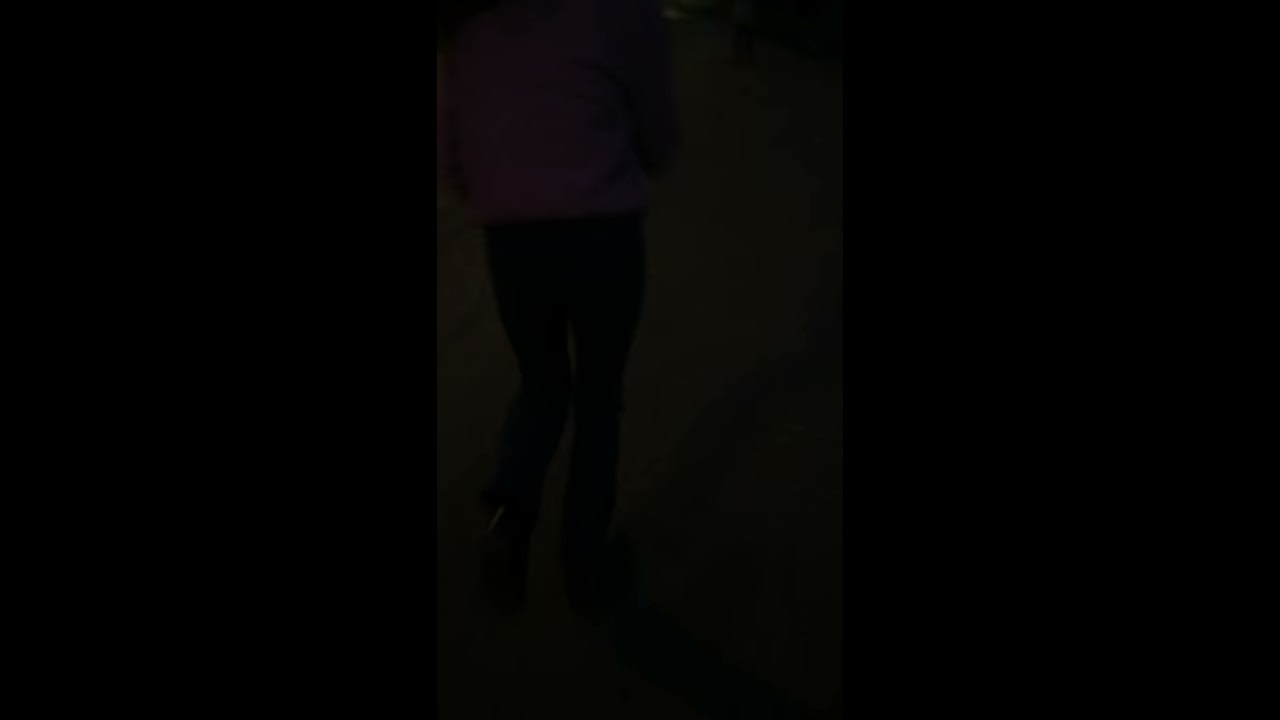In this image, the predominant feature is an almost entirely black background, making it very dark and challenging to discern details. However, at the center of the picture, there appears to be a figure—potentially a person—walking away from the camera. The figure's upper body, waist, legs, and feet can be faintly made out, suggesting possibly a male figure due to the physique. The person is wearing black pants and a pink jacket or sweater. The left leg is slightly lifted off the ground, indicating a walking motion. Despite the obscurity, the figure seems to be in a hallway, and the lack of lighting further complicates the clarity of the image.